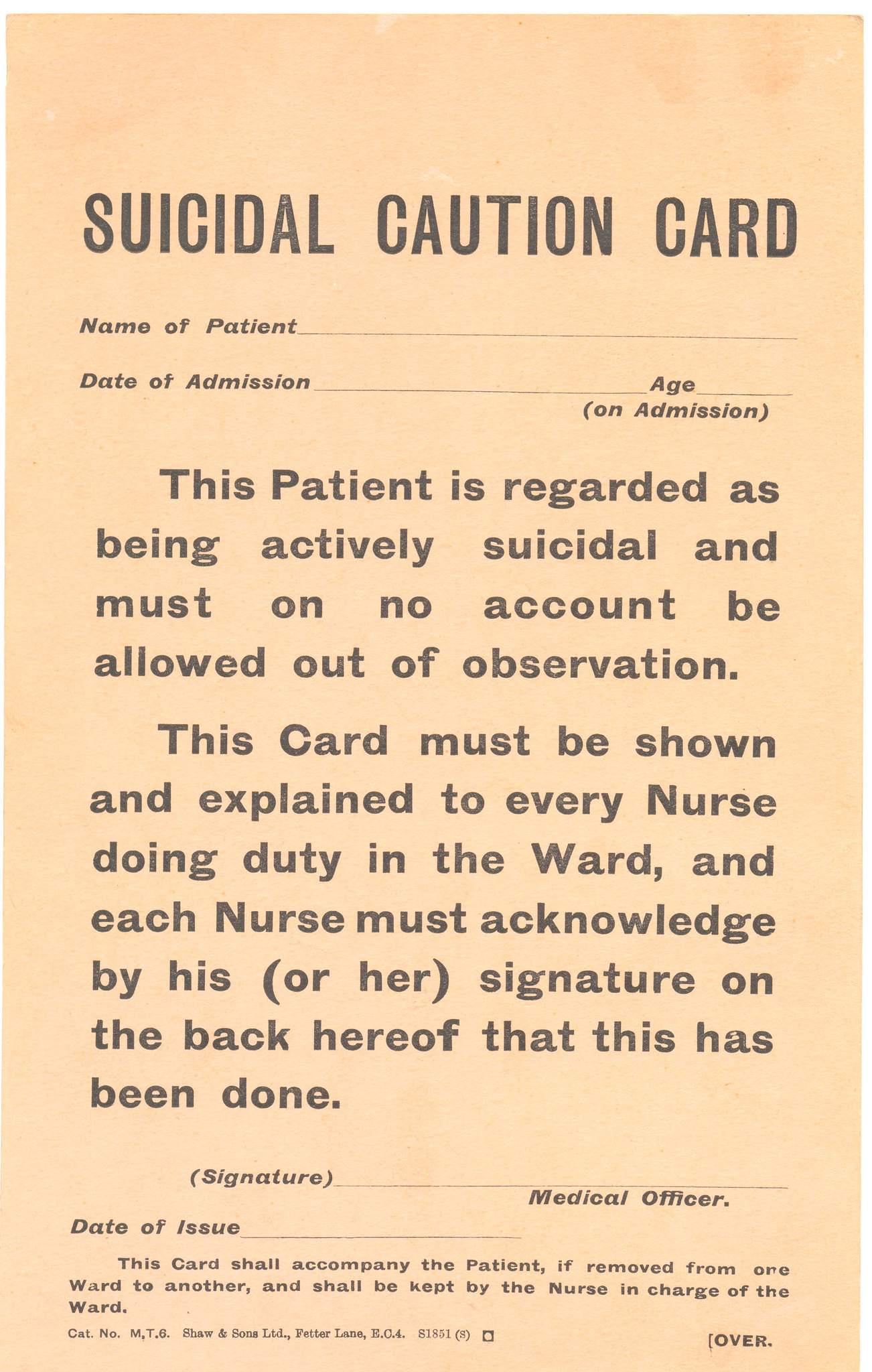This image depicts a "Suicidal Caution Card" used in hospitals to alert medical staff about a patient who is regarded as actively suicidal. The card includes blank spaces to fill in the patient's name, date of admission, and age at the time of admission, none of which are filled out in the image. The card prominently states that the patient must under no circumstances be allowed out of observation. It also has a procedural mandate that the card must be shown and explained to every nurse on duty in the ward, with each nurse required to acknowledge this by signing on the back. Additional spaces exist for a medical officer's signature and the date of issue, both of which are also unfilled. The card is to accompany the patient if they are moved from one ward to another and must be kept by the nurse in charge of the ward. The card serves as a critical reminder to ensure continuous monitoring and strict adherence to safety protocols to protect the patient's well-being.